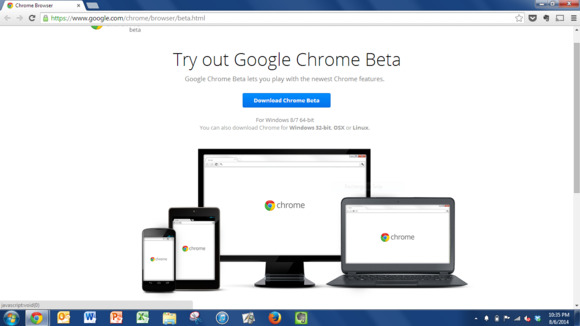In this screenshot of a Google Chrome browser homepage, we see a detailed view of a typical Windows desktop environment. At the bottom of the screen are various icons in the taskbar, starting from the left: the Start button, Google Chrome, Microsoft Word, Microsoft PowerPoint, Microsoft Excel, a Folders tab, iTunes, Mozilla Firefox, and several other unidentifiable icons. 

On the bottom right, the system clock indicates it is 9:15 PM, and the date, though slightly blurry, appears to be August 6, 2014. 

The main browser window features the Google homepage. At the top of the page, there is a promotional banner text that reads, "Try out Google Chrome Beta. Google Chrome Beta lets you play with the newest Chrome features." Below this text, a prominent blue button invites users to "Download Chrome Beta for Windows 8, 7, and 64-bit."

Further down the page, there are images of four different devices— a smartphone, a tablet, a computer monitor, and a laptop—all displaying the Chrome logo on their screens, illustrating the cross-platform compatibility of the browser.